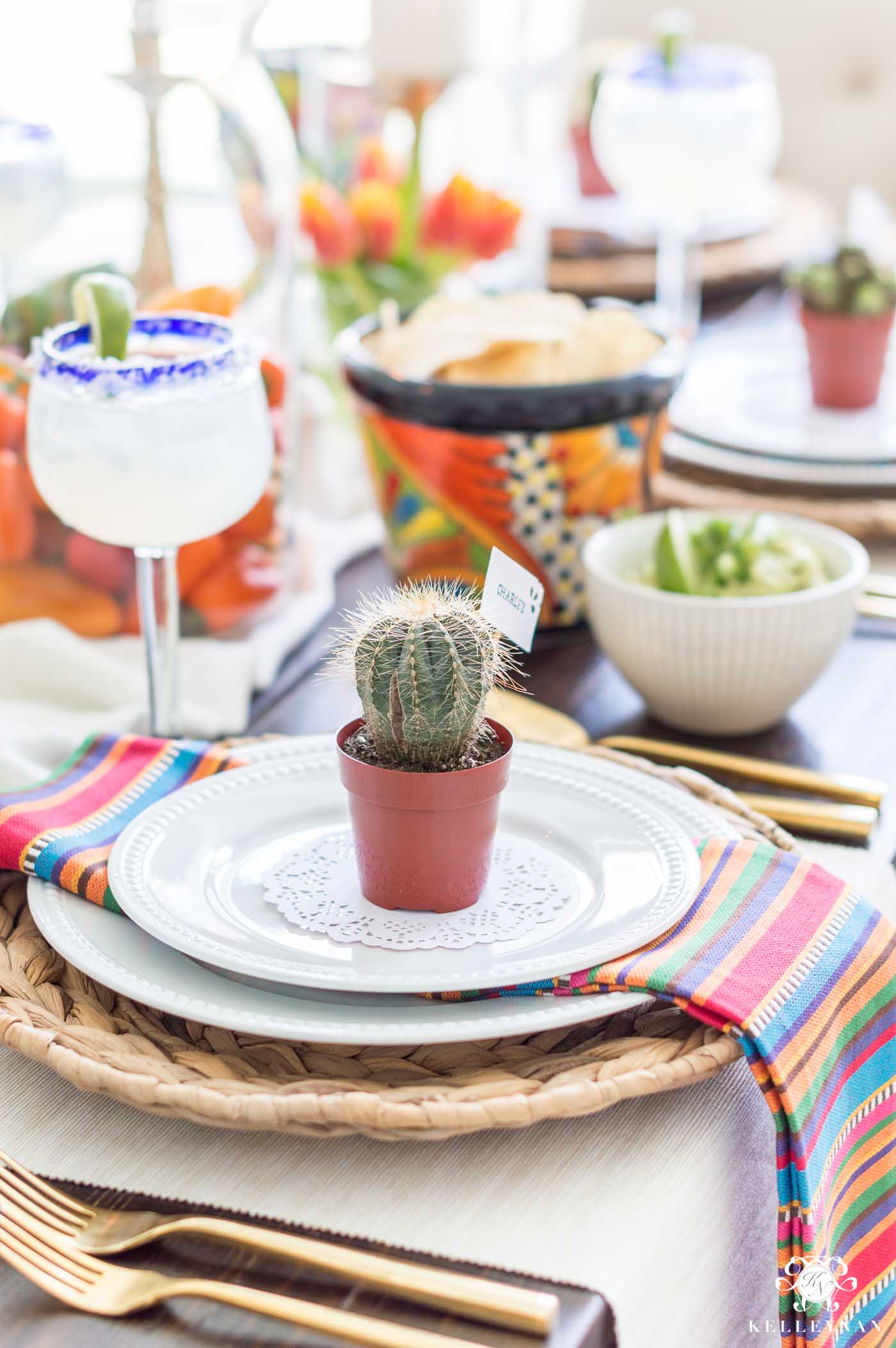The image displays a carefully set white table positioned near the lower center of the frame, showcasing an intricate arrangement of dining elements. At the forefront lies a layered ensemble of plates: a smaller white plate placed atop a larger white ceramic plate, both seated on a tan wicker plate. Beneath this arrangement, a vibrant rectangular napkin with multicolored stripes in orange, green, black, blue, tan, red, yellow, and purple is visible. This setup rests on a dark wooden table.

The place setting features gold dining silverware, with two gold forks on the left and spoons on the right. Atop the layered plates sits a white doily, upon which a red plant holder cradles a green cactus, adding a touch of natural decor.

In the background, on the left side, there is a clear margarita glass with a blue rim, suggesting an alcoholic beverage, garnished with a slice of lime and salt on the rim. Meanwhile, on the right side, a vibrant potted plant resides, its pot adorned with a blend of colors like orange, green, and yellow. The blurred background reveals additional tableware, including more wine glasses and bowls with vivid designs, emphasizing the overall southwestern motif of the setting.